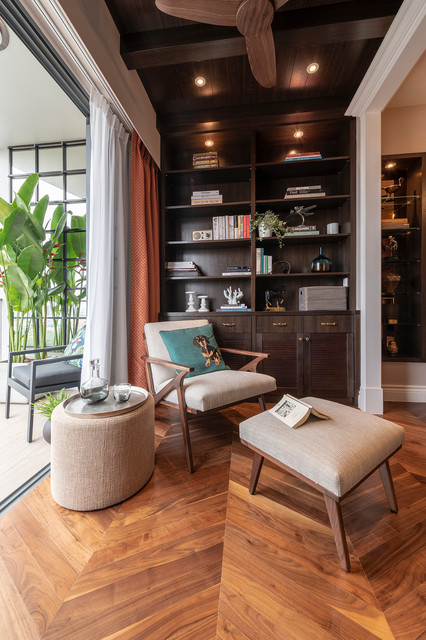This indoor daytime photograph captures a well-decorated living space featuring polished V-shaped wooden floors. Starting in the lower section of the image, there is a beige chair with a wooden frame positioned centrally, adorned with a blue throw pillow showcasing an image of a brown and black dog. In front of the chair is a matching footrest, on which an open book rests. 

To the left of the chair, a cylindrical wooden stool holds a platter with a glass and a carafe. The back of the room is dominated by a dark brown bookshelf spanning from the floor to the ceiling, filled with books, plants, and various knick-knacks. Just below the bookshelf, there are cabinets and drawers for additional storage.

On the right side of the photograph, an opening leads to an adjacent room. On the left, a large sliding glass door or window opens up to a patio area, partially concealed by gray and orange curtains. This outdoor space includes a gray chair and a tall green plant, allowing natural light to flood into the room. Above, the ceiling is made of dark brown wood, equipped with recessed lighting and a brown ceiling fan, completing the warm and stylish aesthetic of the space.